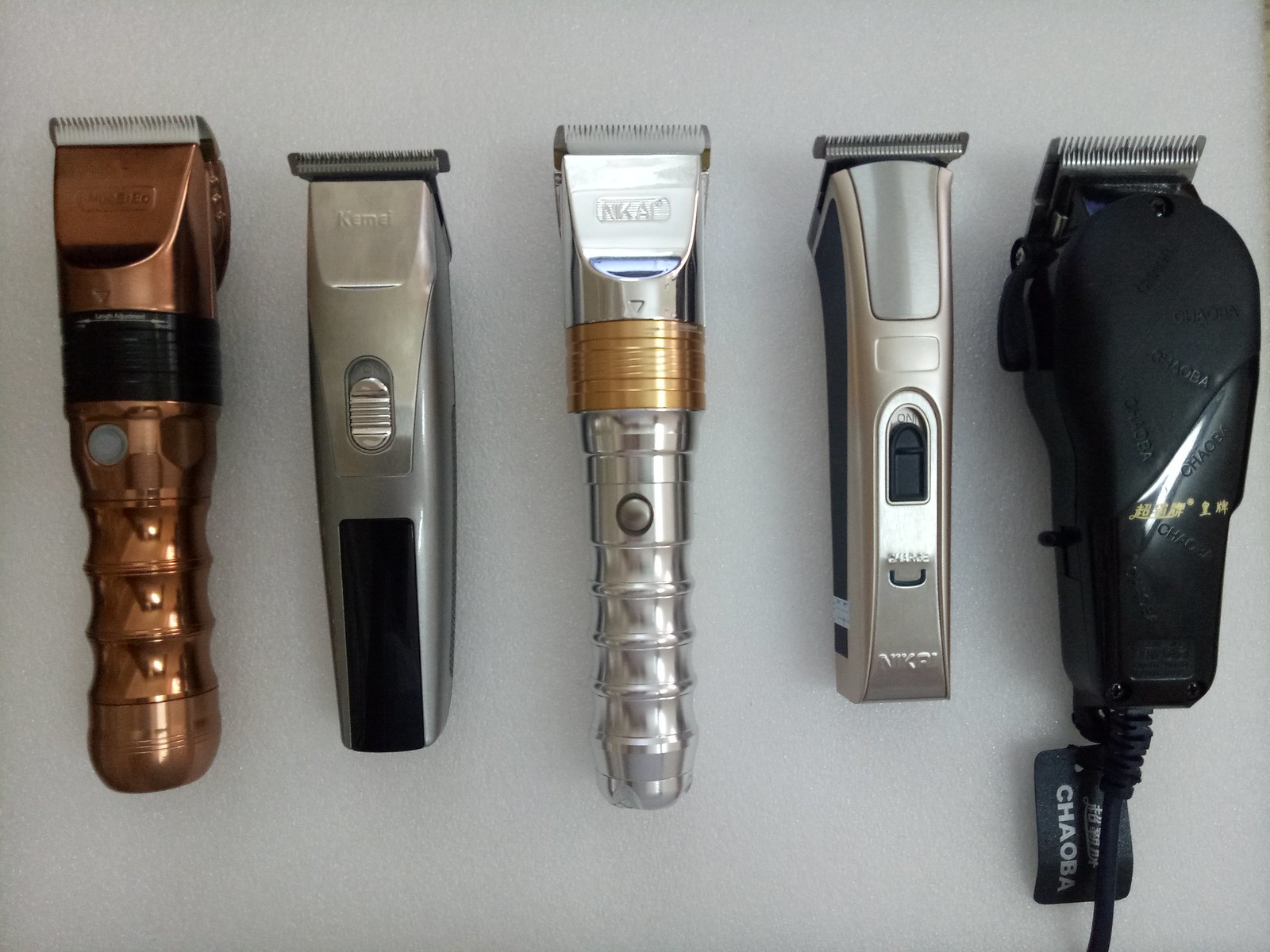This detailed color photograph showcases five different types of electric trimmers, neatly lined up in a row on a light gray surface. The razors, laying horizontally, are the focal point of the image and take up most of the visual space. The trimmers, varying in design and color, exhibit a range of metallic shades including gray, gold, silver, and black. 

Starting from the left, the first trimmer is brassy with a black strip running down the middle. The second trimmer features a mostly silver body with a black handle. Centrally placed is a particularly shiny silver trimmer distinguished by a slender, fluted handle and a gold band around its middle, resembling a microphone in shape. Next, a matte silver trimmer with a small black button in the center stands out. The final trimmer on the far right is predominantly black with some gold lettering and features a visible black cord, indicating its need to be connected to an outlet. 

All five trimmers lack protective guards on their blades, revealing the cutting edges. They are arranged on the gray surface such that each is slightly tilted downwards towards the left, creating a dynamic composition in the photograph.